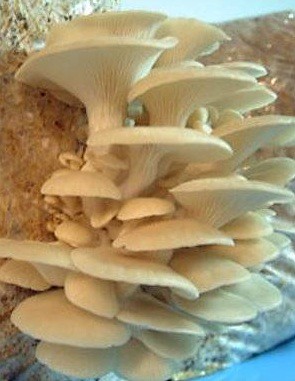This close-up photograph captures a dense cluster of off-white to beige-yellow mushroom-like structures, possibly coral or a type of fungus, layered intricately atop a concrete-like rock formation. The image showcases approximately 15 of these organisms, all bunched together with their vertical stems protruding from the rock and fanning out into flat, thin-rimmed caps. The detailed vertical lines on the stems are clearly visible, emphasizing their structured texture. The mushrooms vary in size, with smaller heads at the base, gradually increasing in size towards the top. Light enters from the top right, casting slight shadows beneath the caps. In the background, there's a blur of turquoise blue in the bottom right corner and light blue at the top, contributing to an ambiguous aquatic or wooded setting. The entire composition fills most of the photo, with no discernible text present.